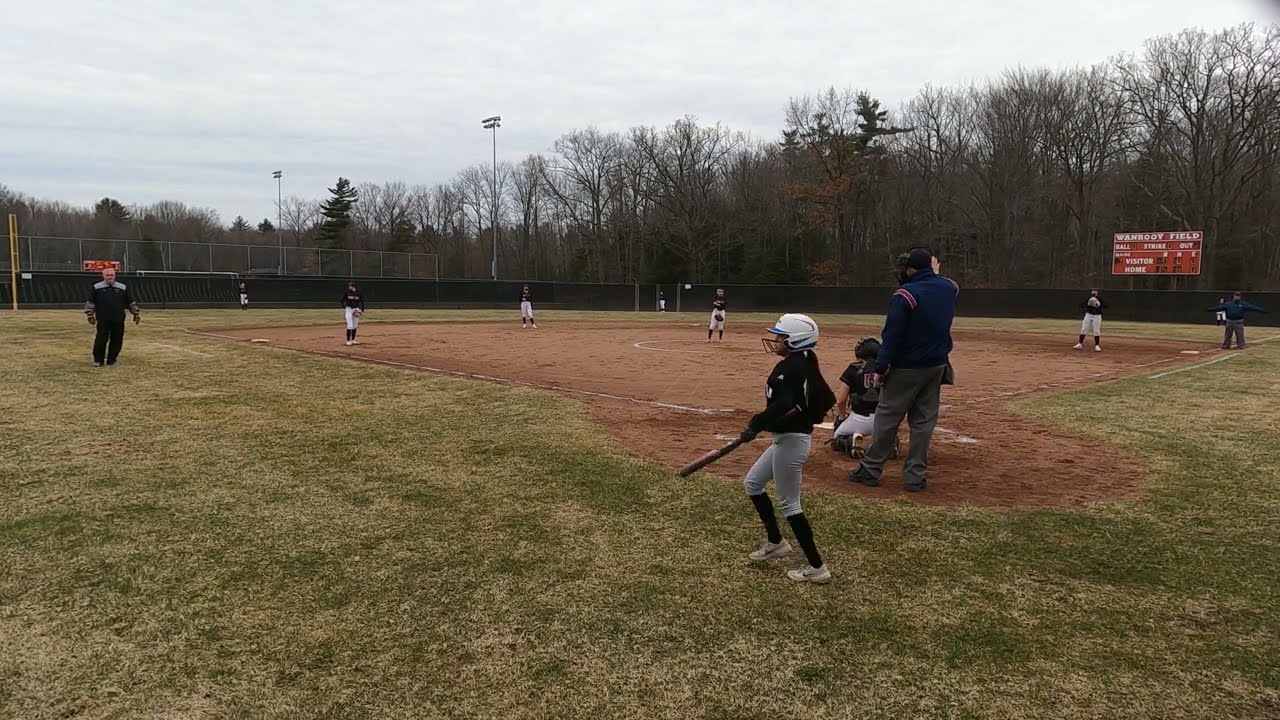The photograph captures a baseball game in progress on a grassy, sage-green field under a gray sky, suggesting a cold fall or winter day. Central to the image, a girl wearing a white helmet, black shirt, white pants, long black socks, and white sneakers is walking up to the plate, holding a baseball bat in her left hand. The umpire, wearing a blue jacket with red stripes over the shoulders, a black helmet, and gray pants, stands at home plate. A black fence surrounds the field, and large stadium lights are visible in the background. Players occupy each base and the outfield, with a man on the left of third base likely serving as the coach. In the distance to the right, a red scoreboard and barren brown trees can be seen. The scene features predominantly green, brown, black, and gray hues, enhancing the chilly and muted atmosphere of the setting.